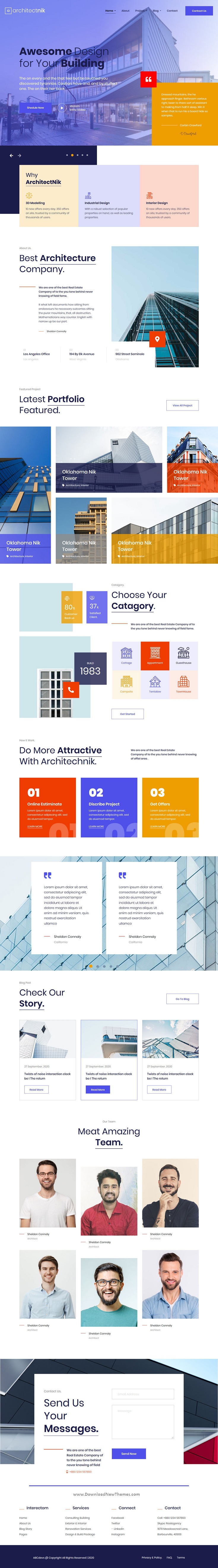This image seems to be a blurry screenshot, possibly of a travel website’s homepage. The layout showcases various travel-related elements and follows a specific structure:

1. **Banner Image Across the Top**: A banner spans the top of the page showing a building or hotel, albeit unclear due to the blurriness.
2. **Bottom Right Corner**: An orange rectangle stands out, likely a button or call-to-action.
3. **White Box Section**: Directly below the banner, there's a white box with a distinct layout.
   - **Top Segment**: Divided into three color-coded areas—peach, blue, and pink.
   - **Left Side**: Contains textual information.
   - **Right Side**: Includes a photo, possibly depicting a bridge with a railing.
4. **Four Outdoor Images**: Below the white box are four side-by-side images, each showcasing different outdoor destinations.
5. **Two Subsequent Sections**: These are followed by two more content sections, details of which are not clearly visible.
6. **Three Colored Bars**: Red, blue, and yellow bars appear next in the vertical layout.
7. **Lower Banner with Message Bars**: Another banner features two white message bars.
8. **Photographs and Footer**: Beneath this, there are several photographs of men, ending with an advertisement or informational bar at the very bottom of the page.

Despite the blurriness, the structure suggests a detailed travel-oriented webpage designed to attract and inform potential travelers.